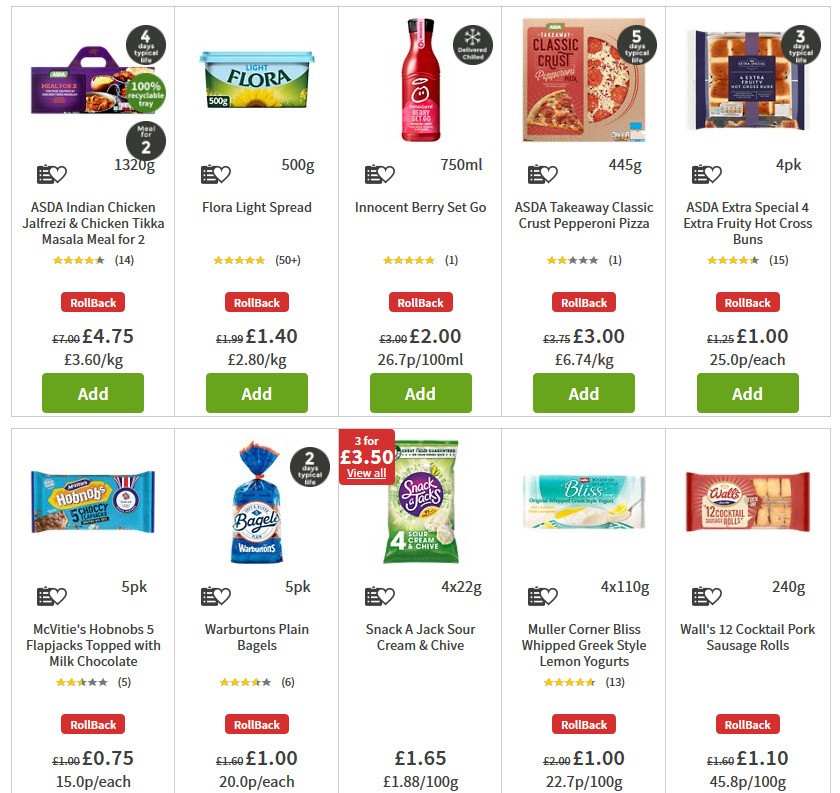Certainly! Here's a cleaned-up and detailed descriptive caption for the image:

---

The image showcases an online shopping platform featuring a diverse array of advertised products, each with distinct visuals and prices displayed in euros. 

Starting from the top left, there is "SDA Indian Chicken Jalfrezi and Chicken Tikka Masala Meal for Two" priced at €4.75. Next to it, the image shows a rolled red bag pattern typical for several products except "Snack-a-Jack Sour Cream and Chive," which features a green pattern at the bottom. 

Continuing, we see "Floral Light Spread" priced at €1.40, accompanied by "Innocent Berry Set Go" at €2.00. Below these items, there is a "Take Away Classic Crust Pepperoni Pizza" costing €3. Following that, "Extra Special and 4 Extra Fruity Hot Cross Buns" are priced at €1. 

Towards the bottom left of the image, we find "McVities Hob Nobs Flapjacks topped with Milk Chocolate" listed at €0.50. Adjacent, there are "World Pattern Plain Bagels" at €1.00, "Snack-a-Jack Sour Cream and Chive" at €1.65, and "Müller Corners Bliss Whipped Greek Style Lemon Yogurt" at €1.00. Finally, the display includes "12 Cocktail Pork Sausage Rolls," priced at €1.10. 

Each product is well-presented, underscoring the variety and affordability of the offerings available on this online shopping platform.

---